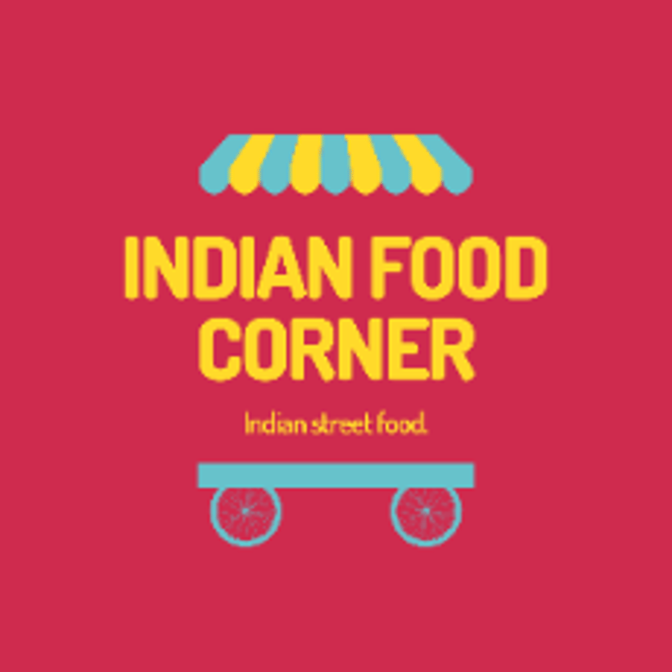The image features a vibrant advertisement for an Indian street food cart, set against a rich red background. Prominently displayed in the center are bold, yellow, capital letters stating "Indian Food Corner," with smaller yellow text below reading "Indian Street Food." Above the text, a striped blue and yellow canopy mimics the classic overhang of a food cart, enhancing the street food theme. Below the text, a detailed illustration of a cart adds to the visual appeal, with its flat base, two wheels complete with blue spokes, all uniformly colored in the same blue shade. The cohesive use of colors and elements effectively captures the essence of an inviting, traditional Indian street food vendor, drawing attention to the vibrant and accessible representation.